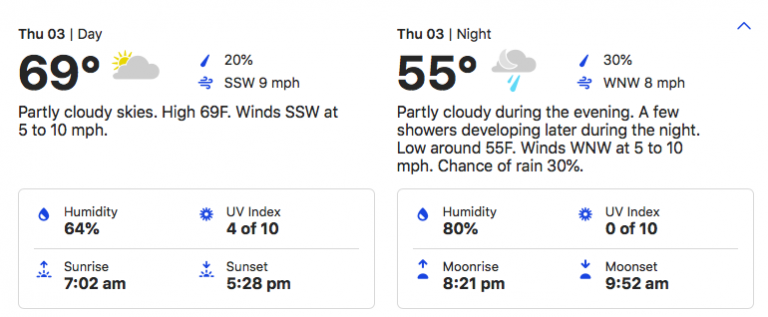This is a detailed weather forecast screenshot, split into two sections for Thursday, the 3rd. The left side showcases the day forecast, while the right side represents the night forecast. 

**Thursday 03 Day:**
- **Temperature:** 69°F (displayed in bold and large font with a small cloud icon)
- **Weather Description:** Partly cloudy skies
- **Humidity:** 64%
- **Wind:** SSW at 5-10 MPH
- **UV Index:** 4 out of 10
- **Sunrise:** 7:02 AM
- **Sunset:** 5:28 PM

**Thursday 03 Night:**
- **Temperature:** 55°F (displayed in bold and large font with a small cloud icon)
- **Weather Description:** Partly cloudy during the evening, with a few showers developing later in the night
- **Chance of Rain:** 30%
- **Humidity:** 30%
- **Wind:** WNW at 5-10 MPH

A series of small weather icons are also displayed to further illustrate the forecast, indicating humidity percentages and wind speeds respectively for day and night.